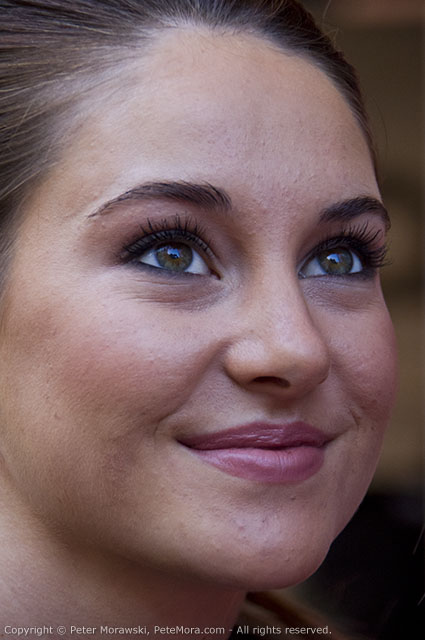The image is a close-up photograph of actress Shailene Woodley, capturing her soft, gentle smile as she looks upward to the top right. She is wearing light pink lipstick, brown eyeliner, and is adorned with make-up that highlights her hazel eyes, which feature a small reflection that appears slightly blue, possibly from the sky. Her dark brown hair is short and pulled back, with brown eyebrows framing her face. Despite a bit of acne on her chin, she appears youthful and composed. The background is a blurry mix of light and dark brown hues, adding to the focus on her facial features. At the bottom left corner of the image, the text reads “© Peter Morosky, PeteMora.com, All rights reserved.”